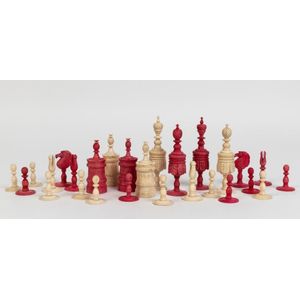This image features an array of chess pieces meticulously arranged against a stark gray background. The pieces are primarily colored in rich reds and a beige-ish, ivory tone. Starting from the left, there are smaller pawns with their distinct round tops. As you move toward the center, the pieces transition to include the larger and thicker bishops, identifiable by their round tops with a cross. Centrally located are the imposing King and Queen; the King is distinguished by his crown with a cross, while the Queen boasts a rounder top adorned with a crown. On the far right, more pawns line up alongside some miscellaneous pieces, completing the set. This detailed arrangement showcases the varied and intricate designs of the chess pieces in a unified and elegant composition.